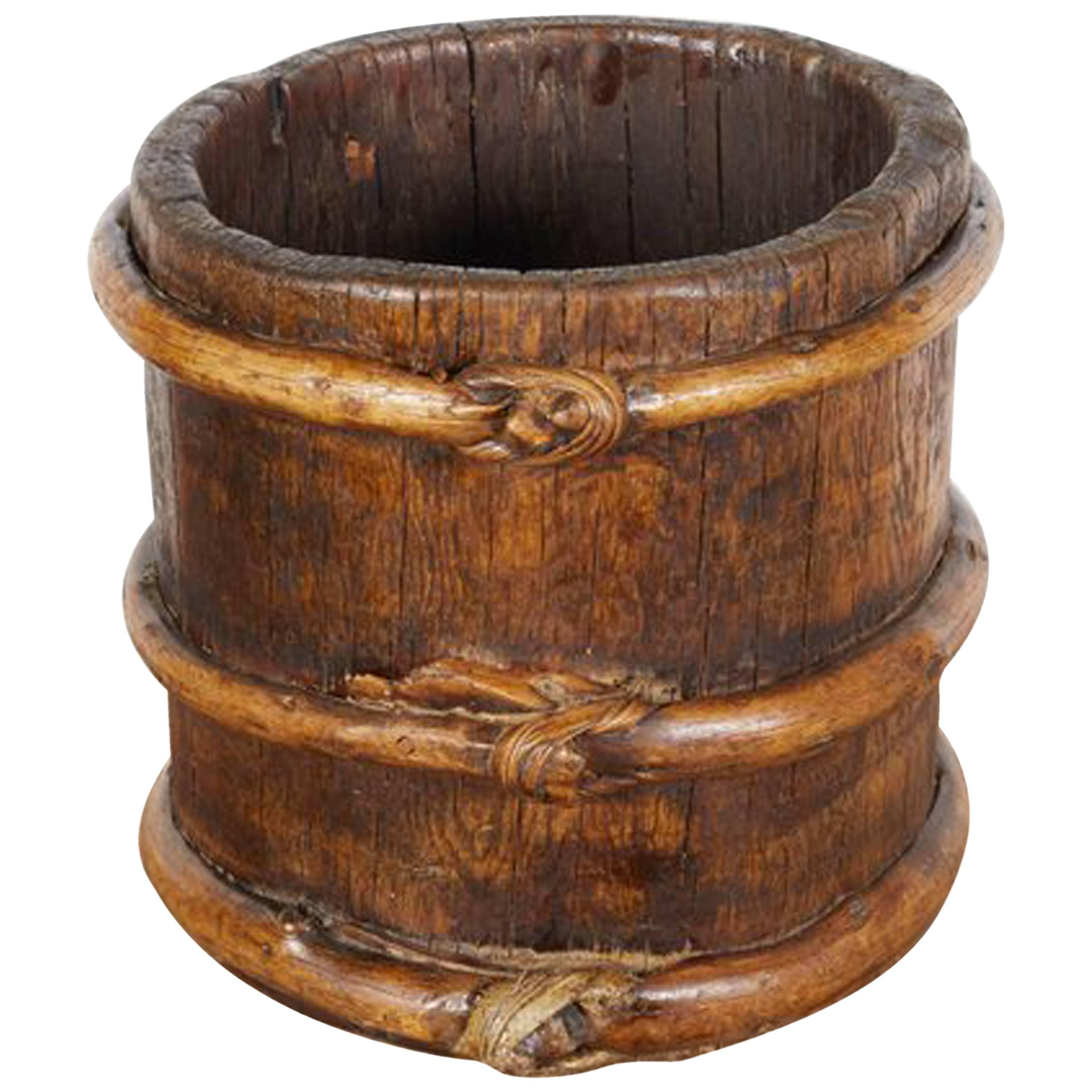The image depicts a well-crafted, hollowed-out wooden object, likely a napkin holder or container of some kind. The piece appears to be made from a single trunk of wood, meticulously stained and protected with a rich, glossy lacquer finish. Its vertical orientation and round shape are accentuated by three distinct wooden bands encircling it—one at the base, one centrally, and one near the top. These bands are seemingly bound with grass or bamboo strings, providing a rustic touch. The surface showcases the natural cracks and textured grain of the wood, suggesting both age and craftsmanship. Small, indeterminate emblems, possibly depicting figures, adorn each ring, adding to its antique aesthetic. The varying shades of light, medium, and dark brown highlight the intricate details and treatment of the wood.